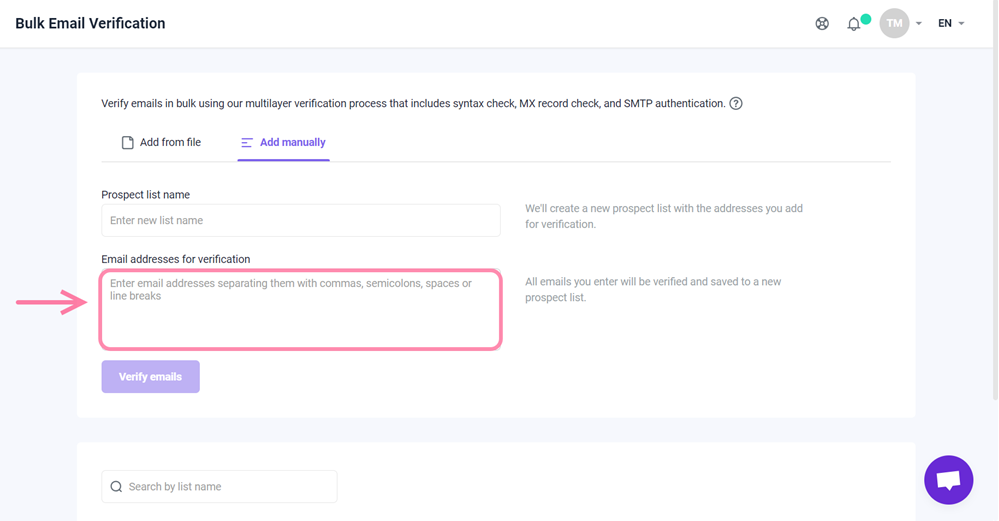This image is a screenshot capturing a user interface for bulk email verification. Central to the screenshot is a red box framing several email addresses that are undergoing the verification process, likely highlighting the status or issue with these specific entries. A red arrow points to this section, drawing immediate attention to it. The screenshot also contains a significant amount of small, somewhat illegible text, presumably containing details relevant to the email verification task. 

In the top corner of the interface, a green notification bell icon is visible, indicating notifications or alerts that have been received. Additionally, a purple chat button is shown, likely providing a support or help chat function for the user. The overall context suggests that the person depicted is engaged in manually verifying a bulk list of email addresses, a task which, while not entirely familiar to the caption provider, is a detailed and meticulous process.